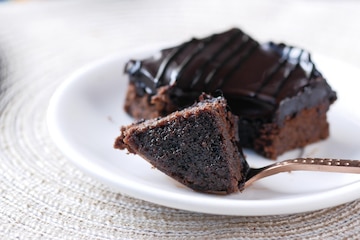The image depicts a richly detailed chocolate dessert, potentially a brownie or a slice of chocolate cake, adorned with a generous layer of dark chocolate fudge and intricate diagonal lines of even darker chocolate. The dessert rests on a gleaming white porcelain plate, placed atop a tan or beige woven table mat. A copper-colored fork with a textured handle, resembling braille, sits beside the dessert, having scooped out a portion that remains uneaten. The background of the image is bright and washed out, highlighting the focal points of the delicious treat and its elegant presentation.